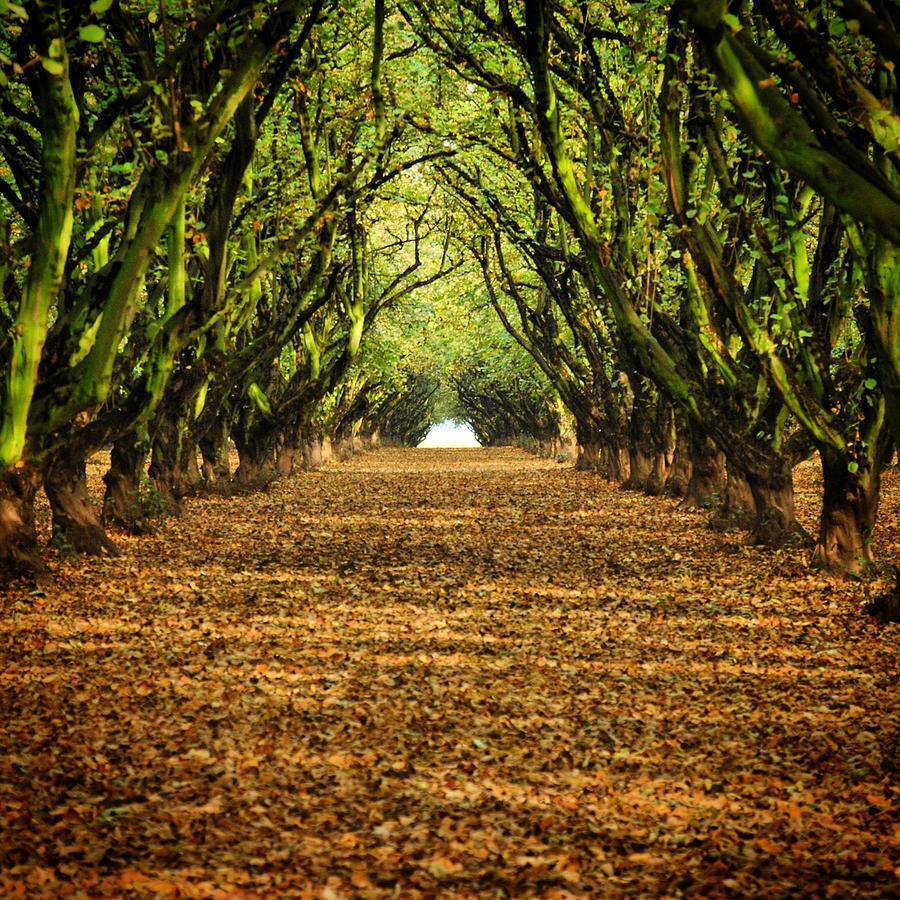The image depicts a serene, leaf-covered trail flanked by rows of trees on both sides. The base of the trees is brown, while the branches and trunks sport a greenish hue, decorated with a touch of hanging greenery. The trail, carpeted with a dense layer of leaves in various shades of dark brown, light brown, and dark orange, stretches far into the distance. Approximately one-third up the trail, the trees on the left appear lined up in a neat row, mirrored by corresponding rows on the right, creating an impression of symmetry. The foliage thickens towards the end of the trail where the trees arch inward, forming an almost cave-like canopy. In the center of the image, a bright white light shines through the opening at the trail's end, framed by the enclosing trees, adding a sense of depth and mystery to the scene.